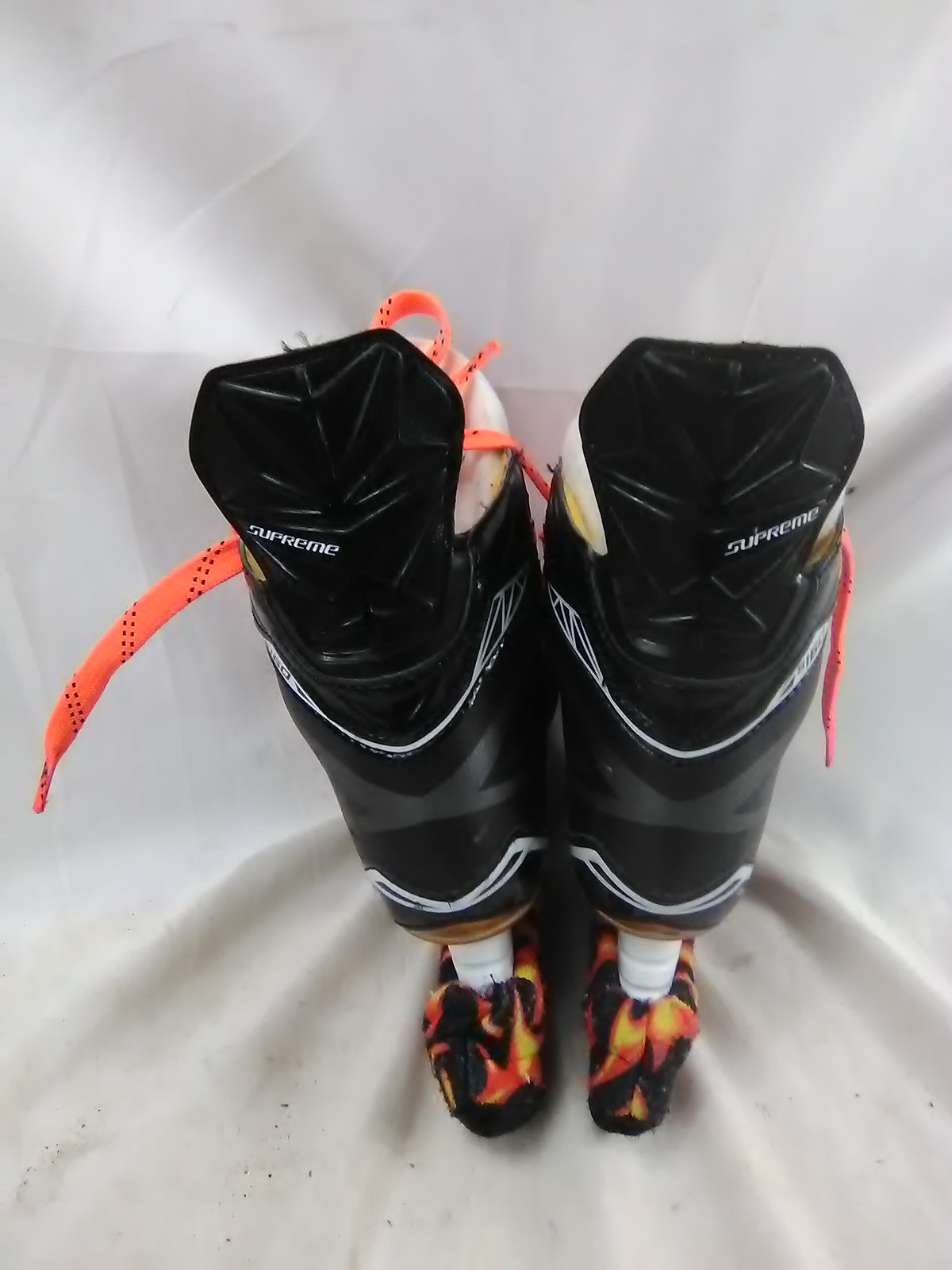The image depicts a pair of black, high-top ice skates positioned on a white blanket or cloth, providing a stark, clean background. Viewed from the back, the skates feature white and gray design elements atop a white heel and an orange-brown bottom. Their distinctive orange and black laces hang partially outwards, with "Supreme" inscribed in white text on the rear. The sole is peculiar; instead of a traditional blade, a rod extends from the bottom, suggesting the blades are covered with a black, orange, and yellow cheetah print cushion. The right skate appears torn on the left side, revealing a yellow and orange sponge-like material inside. The image's lighting highlights subtle variations in the white cloth, displaying shades of gray depending on the light exposure.